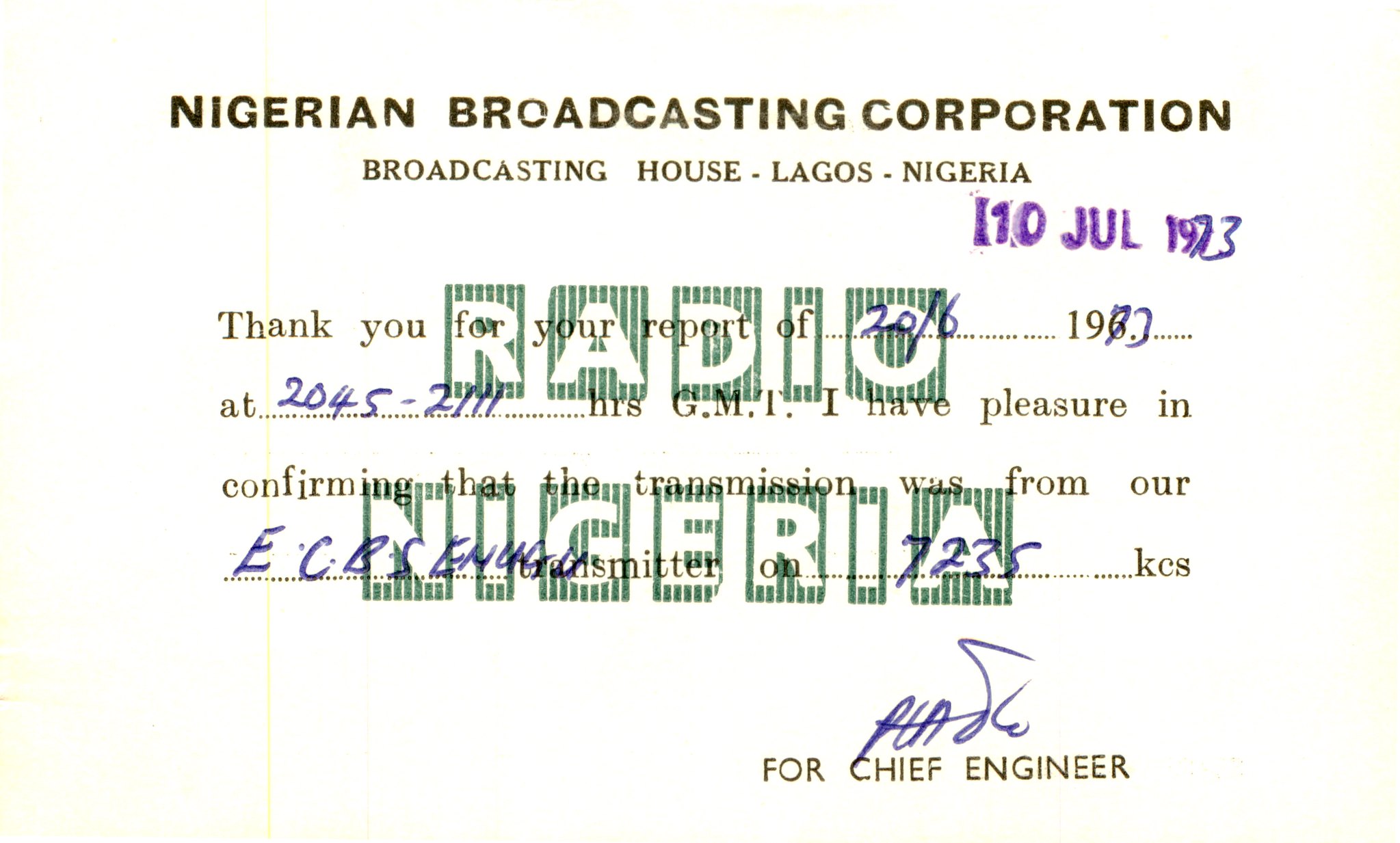The image depicts a document, possibly a radio verification card or a flyer, featuring both printed and handwritten text. At the top, in bold black typewriter font, it reads "Nigerian Broadcasting Corporation," followed by "Broadcasting House, Lagos, Nigeria" in smaller text underneath. A striking purple stamp on the right side states "10th July, 1973," with the date "7-3" written by hand in pen. 

Below this, printed text reads, "Thank you for your report of 2016-1973 at 2045-2111 GMT." This is followed by a confirmation message: "I have pleasure in confirming that the transmission was from our ECBS transmitter on 7235 KCS." It is signed in blue ink with "For Chief Engineer" printed beneath. Adding depth to the document, the background features recurring text "Radio Nigeria" in white, set against green rectangular boxes, contrasting with the bright white-yellowish color of the entire document.